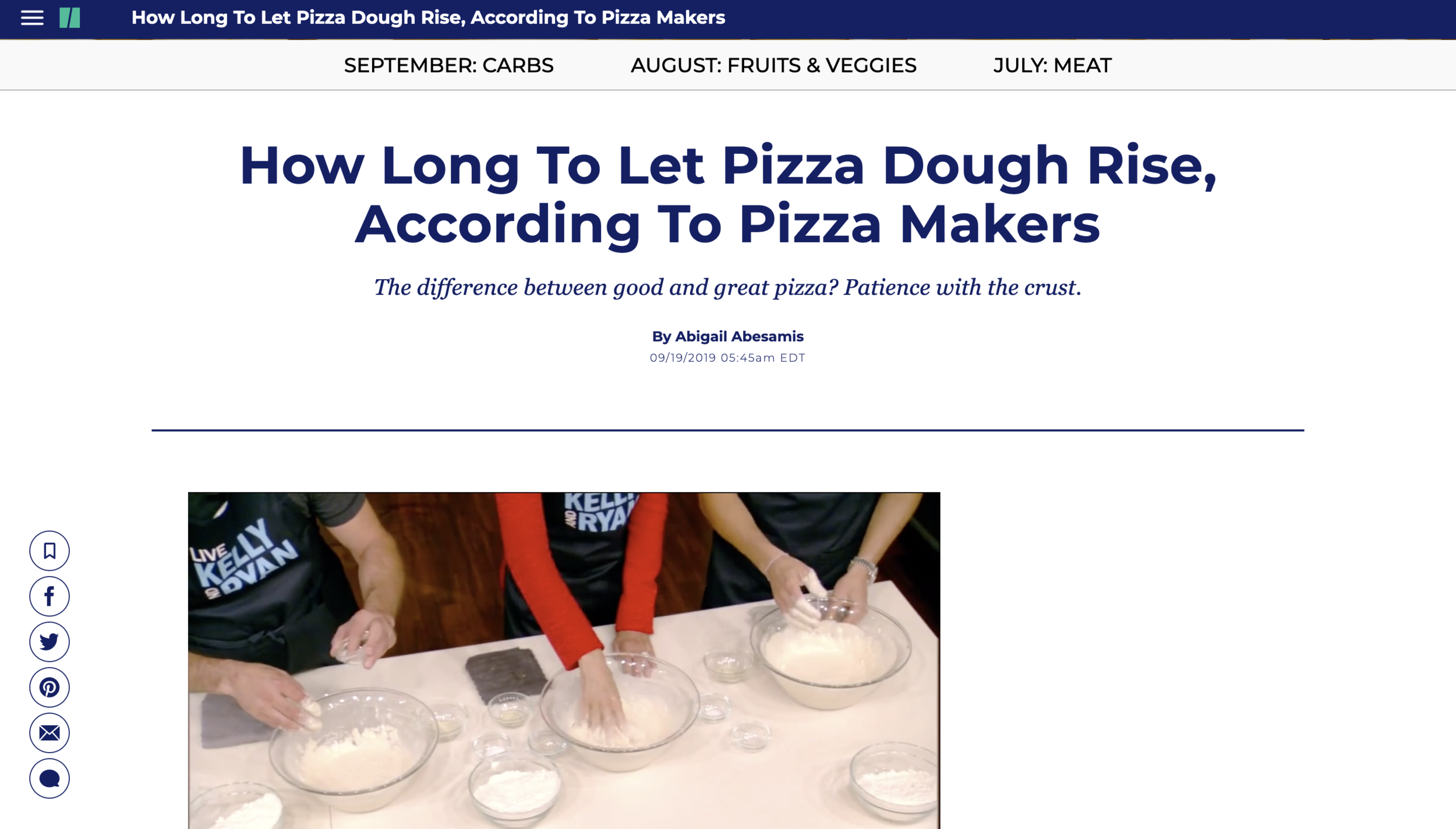In a cozy kitchen setting, three pizza makers sit around a table focused on their craft. On the table, there are three large glass bowls, each containing a brown liquid mixture—likely the beginnings of a pizza dough mixture in the crucial rising phase. Surrounding these bowls are numerous small clear glass bowls filled with various ingredients, including two smaller glass bowls containing white powder, presumably flour or yeast. The scene underscores an essential lesson in pizza making: the key difference between a good pizza and a great one is patience, particularly when it comes to allowing the dough to rise properly. The image captures a moment of quiet dedication, highlighting the meticulous process that is fundamental to crafting the perfect pizza crust.